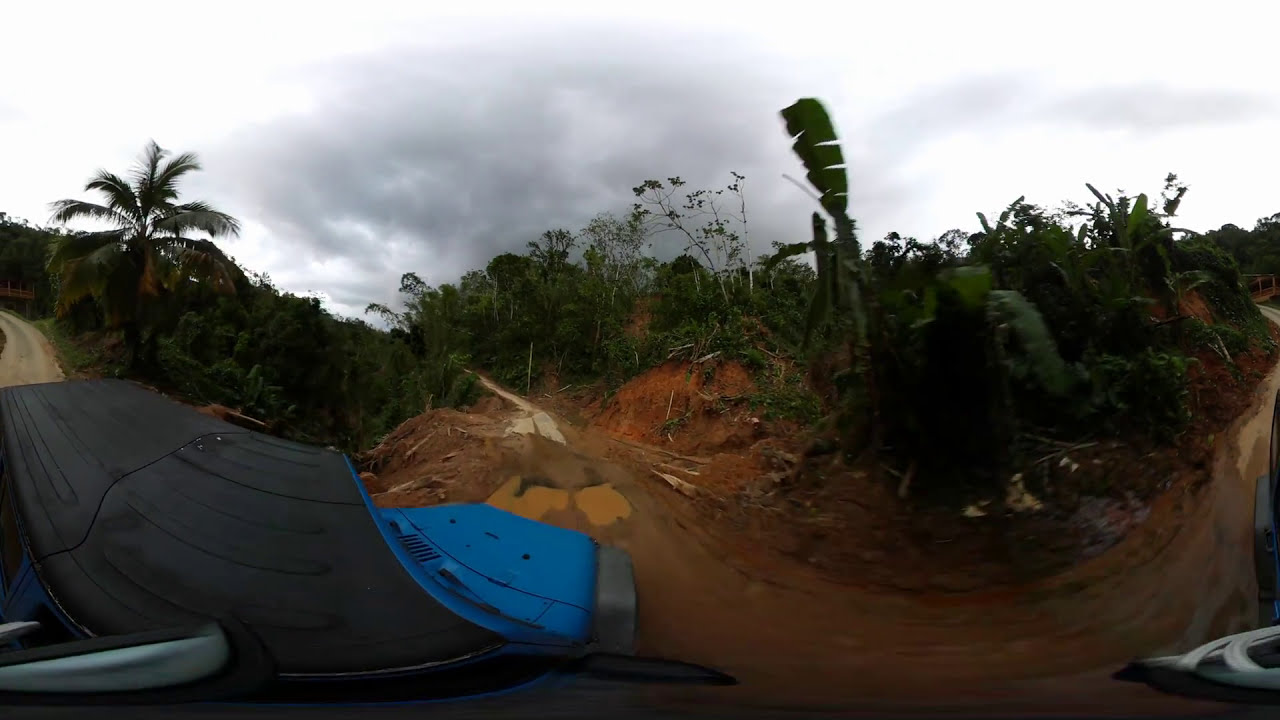A vivid image depicts a rugged, dripping-wet off-road adventure, seemingly captured from a dash cam as a jeep navigates a treacherous, narrow, reddish-brown clay road in Hawaii. The scene, dampened by recent rain, showcases ruts and muddy puddles decorating the path, giving it an unmistakably challenging appearance. Enveloped by lush, dense tropical foliage, including vibrant green shrubbery and towering palm trees, the landscape exudes a wild, jungle-like atmosphere. In the background, a bridge is faintly visible amidst the thick greenery. The sky looms overhead, shrouded in gray, with heavy clouds suggesting a gloomy, sunless day. The jeep, with its black and blue exterior, stands out as it ventures through this vibrant yet foreboding terrain, symbolizing both adventure and the raw beauty of nature. In the bottom left corner of the photograph, a mysterious structure peeks into view, adding an element of intrigue to the rugged scene.